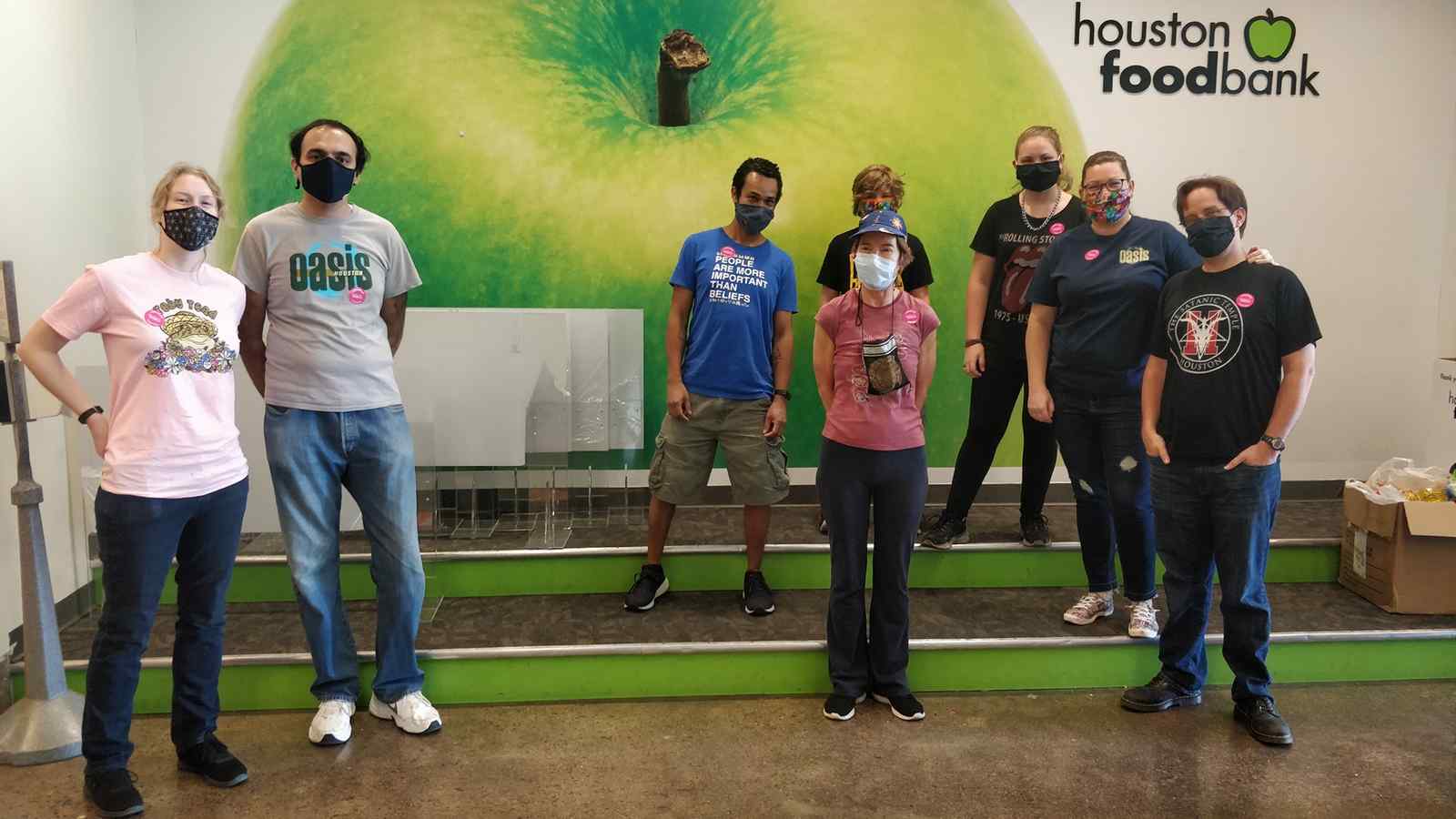This indoor color photograph captures a group of eight people posing in front of a wall adorned with a graphic depiction of a large green apple with a brown stem. The wall, predominantly white, features the words "Houston Food Bank" in bold black text on the upper right, accompanied by a smaller green apple with a black outline. The subjects, who are all wearing face masks, are arranged on two apple-green painted risers and a brown tile floor in front.

From left to right, on the floor, stands a Caucasian woman with blonde hair, wearing a white t-shirt with a graphic design, blue jeans, and black sneakers. Next to her is a balding Caucasian man with dark hair, in a gray t-shirt with a black graphic, faded blue jeans, and white sneakers. In the center of the photograph, a woman in a pink t-shirt, black jeans, and black sneakers is standing on the floor, with a young man in a bright blue t-shirt, khaki cargo shorts, and black sneakers positioned behind her on the first riser. Next to him is a middle-aged blonde woman, partially obscured, in a black short-sleeved t-shirt. On the far right, on the floor, a young man with dark brown hair and a black t-shirt featuring a gold circle graphic pairs his outfit with blue jeans and brown work shoes. Behind him on the first riser stands a young woman with light brown hair, dressed in a dark gray t-shirt, dark blue jeans, and white athletic shoes. Lastly, on the second riser, is a young woman with light brown or blonde hair, wearing a black t-shirt with red and white text, dark blue jeans, and black sneakers. The setting includes two steps with green fronts and dark brown tops leading up to the wall. There is also a box in the right-hand corner of the floor area.